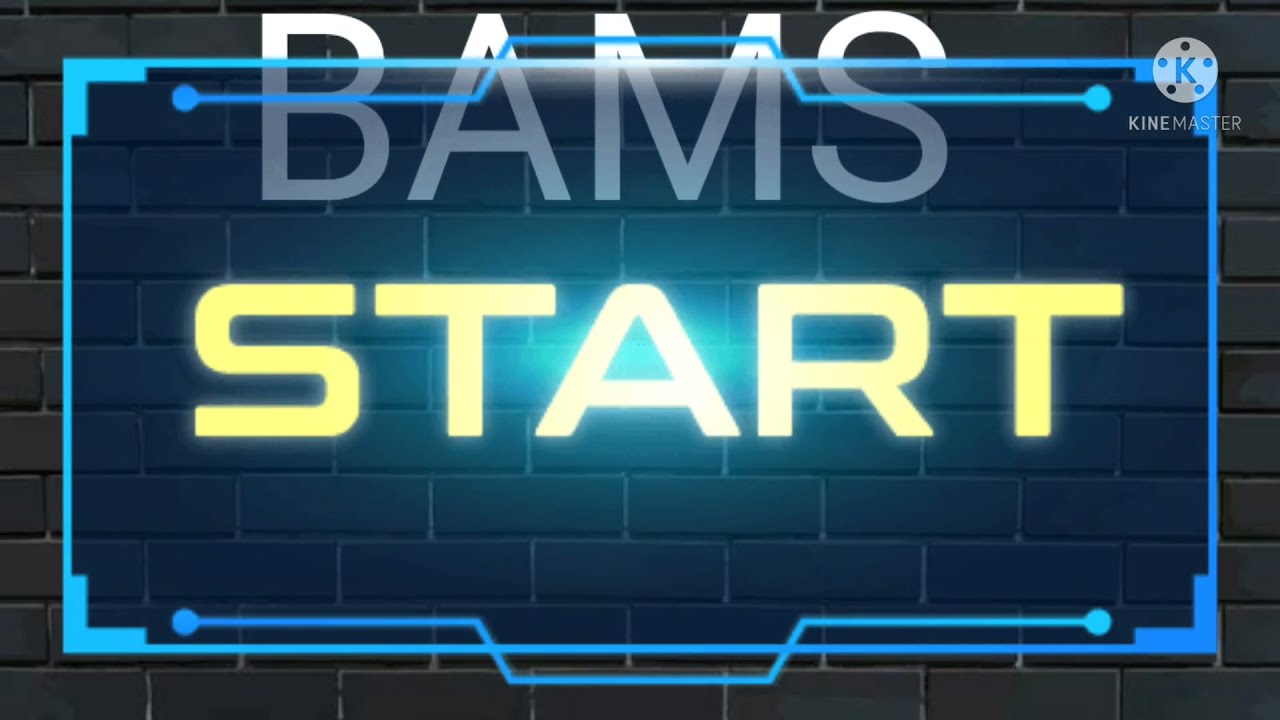The image is a horizontal rectangular frame featuring a black or charcoal-colored brick wall as the background. Dominating the foreground, large all-caps gray letters spell out "BAMS" at the top center, partially enclosed by a blue rectangular outline that extends around the middle and sides of the image. Directly below "BAMS," in the very center, the word "START" appears in large, gold-highlighted letters, with the 'A' particularly illuminated. This blue outline appears digitally stylized, with bends reaching out and small circles on each side. Prominently in the upper right corner, a white circle encloses a large blue "K," beneath which the word "KineMaster" is printed in all-caps gray letters. The overall composition, with its digital and bold elements, suggests it may be a still from a video game or a video production application.